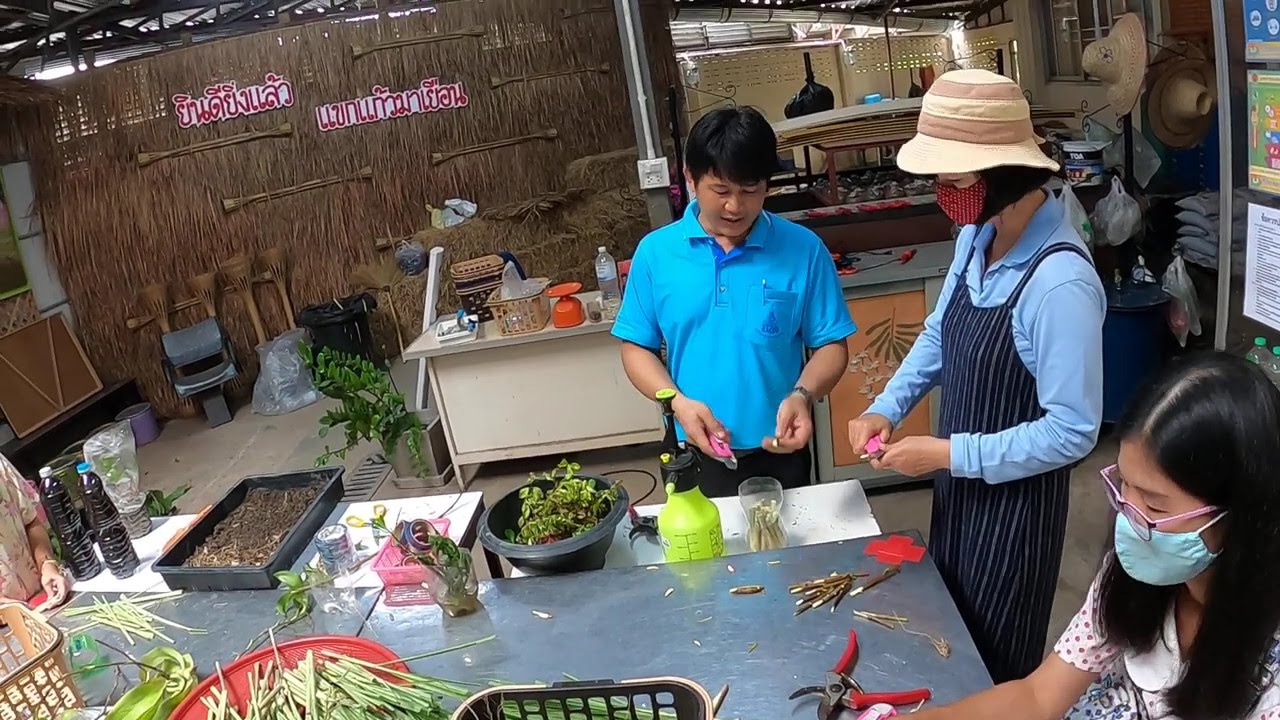The image depicts an Asian gardening workshop where an instructor and participants are learning how to trim and pot plants. Central to the scene is a man in a bright blue shirt, wielding a small knife, who stands over a silver metal table filled with trays and pots. He is teaching a woman in a long-sleeve collared light blue shirt, who is wearing a navy blue striped apron over her outfit and a beige sun hat with brown stripes. She has a red face mask and holds garden shears. Beside her, another female participant with pink glasses, a blue face mask, and a white shirt with polka dots, is seated. The table is laden with gardening tools, including knives and watering equipment, surrounded by various potted plants and cuttings. Straw walls with foreign, likely Asian, language text form the background, and the left side of the image partially shows another woman and two bottles. The overall atmosphere is industrious and educational, with everyone actively engaged in the gardening process.